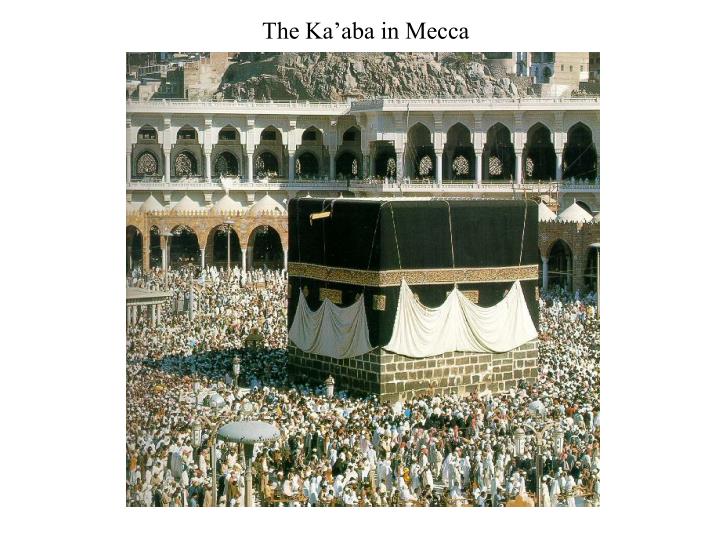The photograph captures the bustling activity at the holy site of the Kaaba in Mecca, as indicated by the black text on a white border at the top of the image. At the center of the scene stands the Kaaba, a large rectangular building with its lower part composed of large square-shaped stones and its upper part painted in black. Surrounding this focal point is a sprawling courtyard teeming with worshippers and pilgrims, many of whom are dressed in traditional white robes and headdresses. The courtyard is encircled by a two-story wall, featuring multiple arches and pillars; the bottom floor is constructed from red bricks while the top floor appears to be made from white stone. The photograph, taken during daylight, highlights the sunlight casting over the massive crowd and the historical architectural elements of the site.